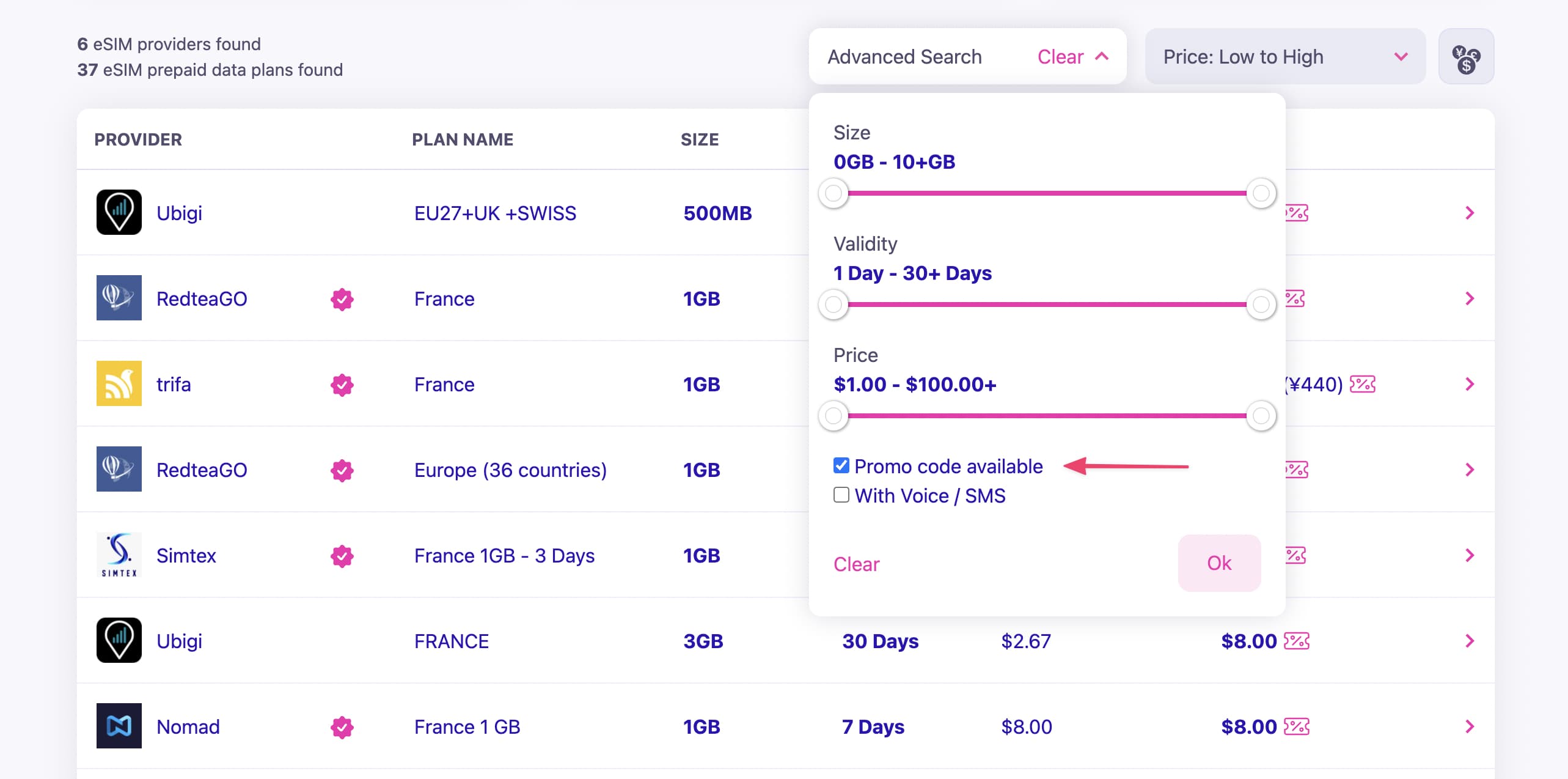The screenshot appears to be from a telecommunication data-sharing website, displaying various data plans offered by different providers. On the far left of the page, providers such as UBI, Trefra, Syntex, and Nomad are listed, showcasing their respective plans. Specifically, the UBI plan offers 500 megabytes per month for a fee that includes an additional cost for URLs in the UK and Switzerland. Similarly, Redtree GO in France and Trefra in France each offer plans providing 1 gigabyte of data.

At the top of the page, there is a navigation bar that includes an advanced search option, allowing users to filter plans based on pricing from high to low. In the search box, users can specify criteria such as data size (10+ gigabytes), validity periods (1 day to 30+ days), and price range ($1 to $100). There is also an option to apply a promotional code, with choices for delivery either digitally or via voice/SMS.

Overall, the site offers a comprehensive comparison of data plans across various telecommunication providers, detailing the data allocations, associated costs, and additional features. The layout enables users to navigate and select the best plan suited to their data needs and budget. The screenshot likely comes from a desktop or laptop display, given the layout and detail visible.